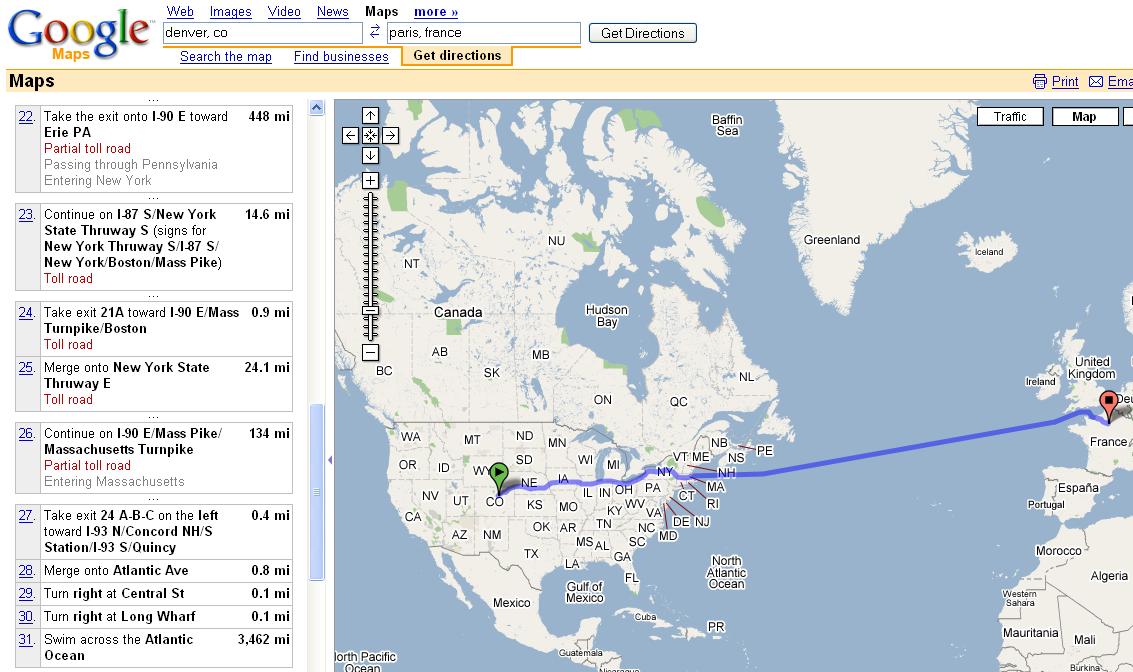The image depicts a Google Maps route from Colorado, USA, to France. The starting point in Colorado is marked with a green bubble and an arrow, while the destination in France is indicated by a red bubble with a marker. The route is visually represented by a blue line tracing the path of travel. The journey takes you through several states including Nebraska, Iowa, Illinois, Michigan (or Indiana), Ohio, a corner of Pennsylvania, and through New York, Massachusetts, and Connecticut. The distance to Pennsylvania alone is 448 miles, while the oceanic portion of the trip spans 3,462 miles. Overall, it's a detailed and lengthy journey from the heart of the United States to Europe.